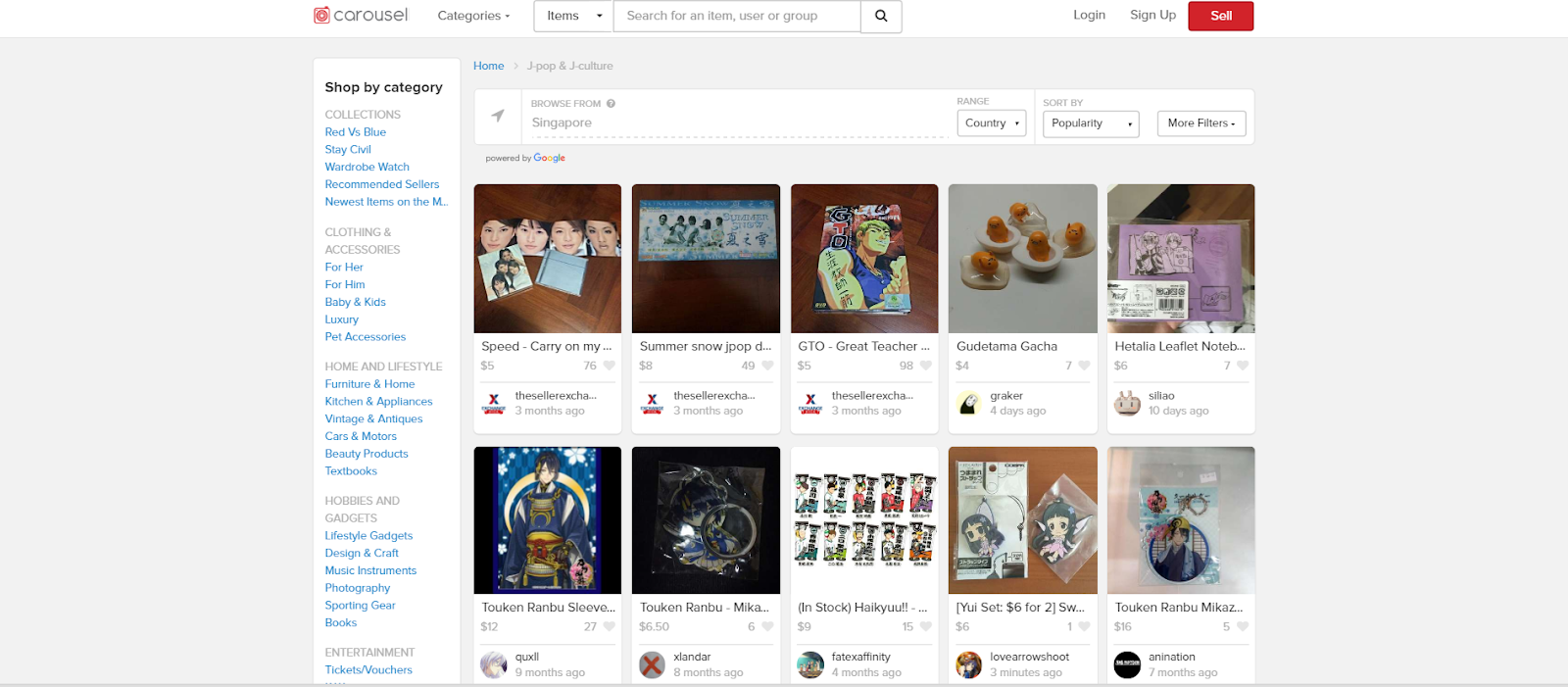The screenshot presented showcases an e-commerce website with various user interface elements and navigation options. At the top is a search bar accompanied by a magnifying glass icon, facilitating keyword searches. Beside the search bar are options to "Login" and "Sign Up", as well as a prominently highlighted "Sale" banner in white text on a red rectangle. 

The website features a carousel of categories titled "Shop by Category" and "Collections," providing an organized view. Each category is presented as a list with blue text, including sections for "Clothing & Accessories", "Hobbies & Gadgets", and "Entertainment", though specific items in these lists are too small to identify clearly. 

Underneath the carousel, users can "Sort by Popularity" or apply "More Filters" to refine their shopping experience. Additionally, the main body of the page displays 10 item listings inside white rectangles. The details in the first rectangle are unclear, but it appears to involve pictures on a table. The second rectangle features a table with another image, and the third one seems to display a magazine.